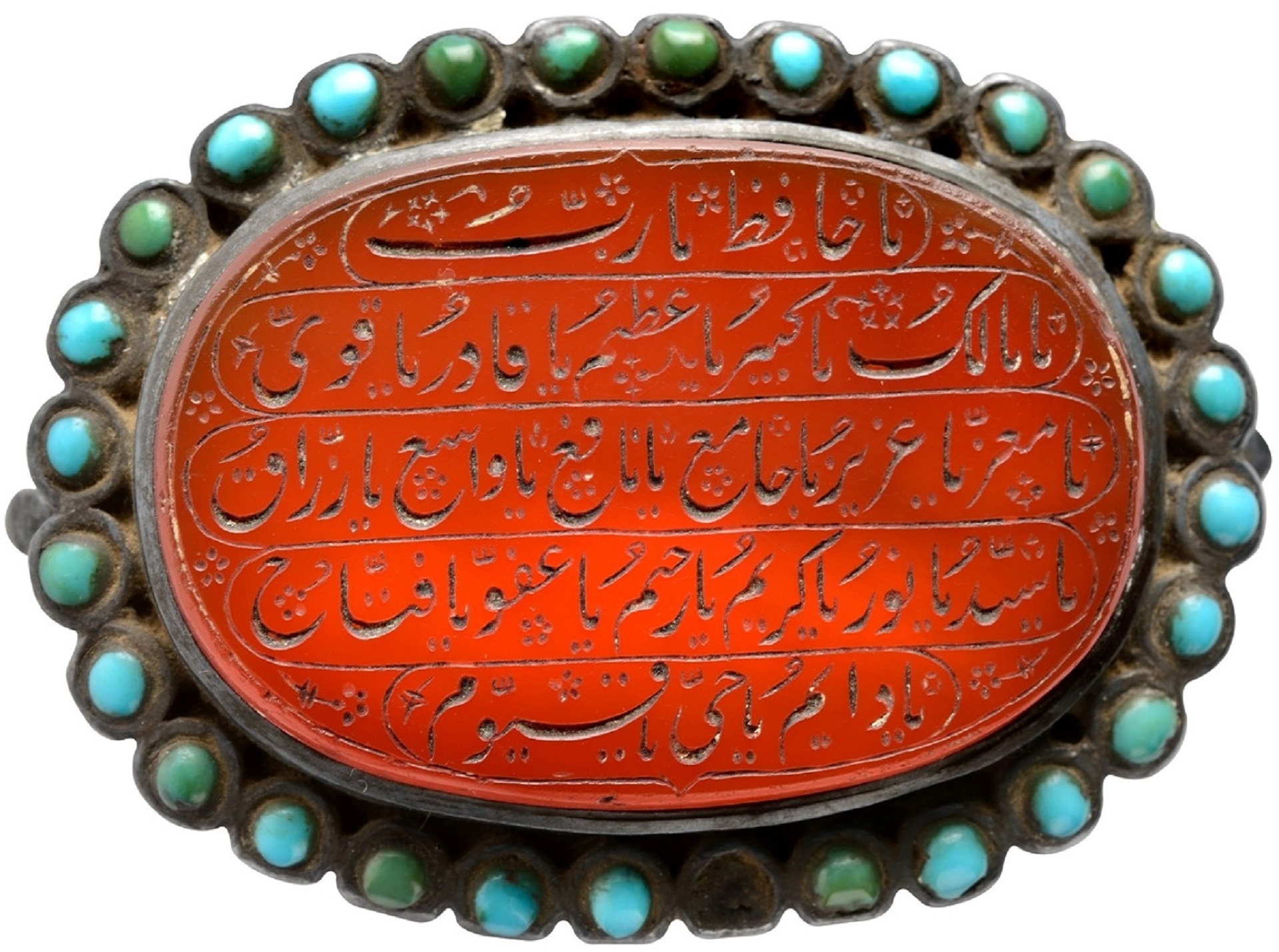The image features a very old, decorative item, likely intended to be worn, resembling a medallion or brooch. Set against a white background, its structure is predominantly made of a silver material that appears tarnished in places. The focal point is an oval-shaped center of a reddish-orange hue, possibly a stone or other solid material, which is intricately engraved with rows of unfamiliar script, potentially Arabic or another Middle Eastern language. Five separate rows of this script are etched within black outlines. Encircling this central area is a silver ring, further bordered by small, embedded blue stones, likely turquoise, interspersed with a few green stones. Some of these are arranged in irregular patterns, such as groups of three or individually spaced, with one turquoise stone conspicuously missing at the bottom. This detailed ornament thus combines elements of tarnished silver, red-orange stone, turquoise, and occasional green stones, showcasing a blend of age, artistry, and cultural mystery.